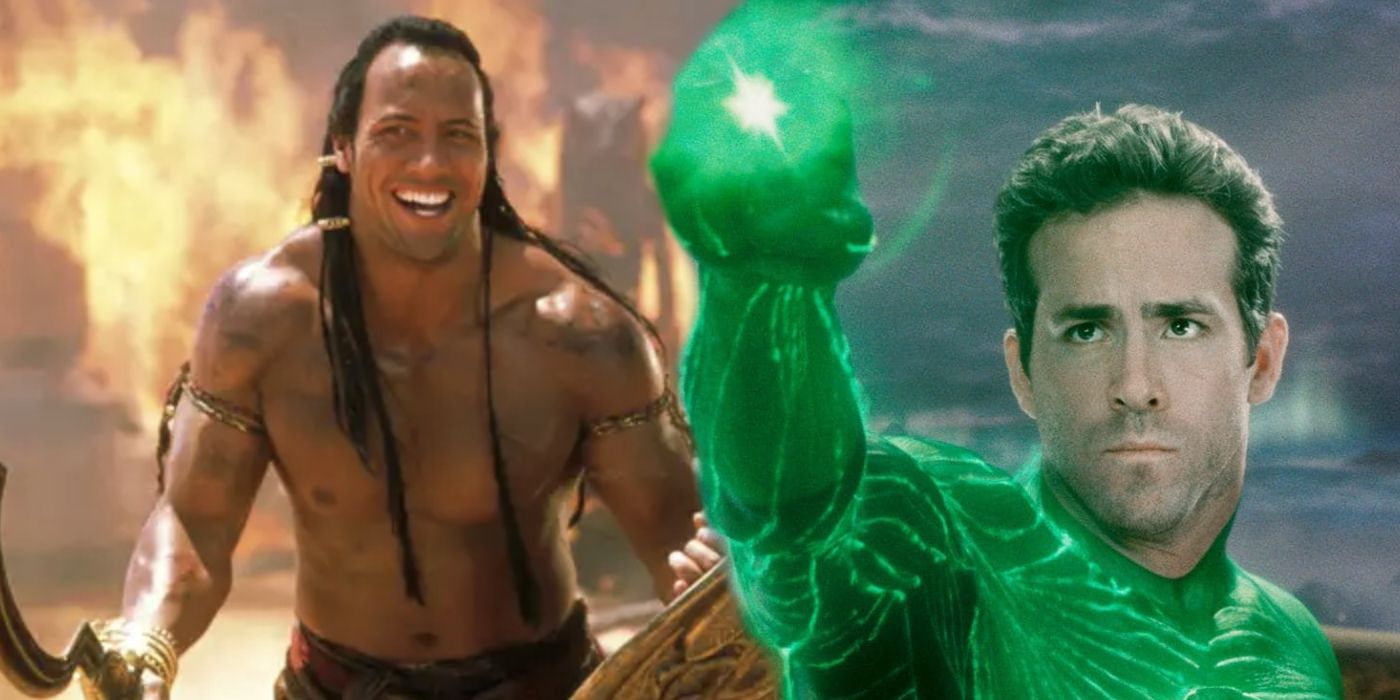The photograph is a dynamic and striking composite featuring two well-known actors, each portraying their respective superhero characters. On the left side, Dwayne "The Rock" Johnson stands heroically amidst a backdrop of roaring flames. He is depicted in a barbaric, gladiator-like costume, reminiscent of Roman or possibly Conan the Barbarian, characterized by his shirtless, heavily muscled torso adorned with gold bracelets and braided hair fastened with gold clasps. He grips a golden shield with his left hand and brandishes a sickle or sword in his right.

On the right side of the photograph, Ryan Reynolds embodies the Green Lantern. Dressed in an vibrant and glowing green suit, Reynolds raises his right fist which is adorned with an illuminated green ring. The background behind him contrasts sharply with Johnson's fiery scene, featuring serene blue and cloudy skies. This juxtaposition highlights not only the differences between their respective movie universes but also the distinct visual styles of their characters. The overall image serves as a crossover advertisement, merging the explosive, intense energy of Johnson's character with the luminous, mystical essence of Reynolds' Green Lantern.